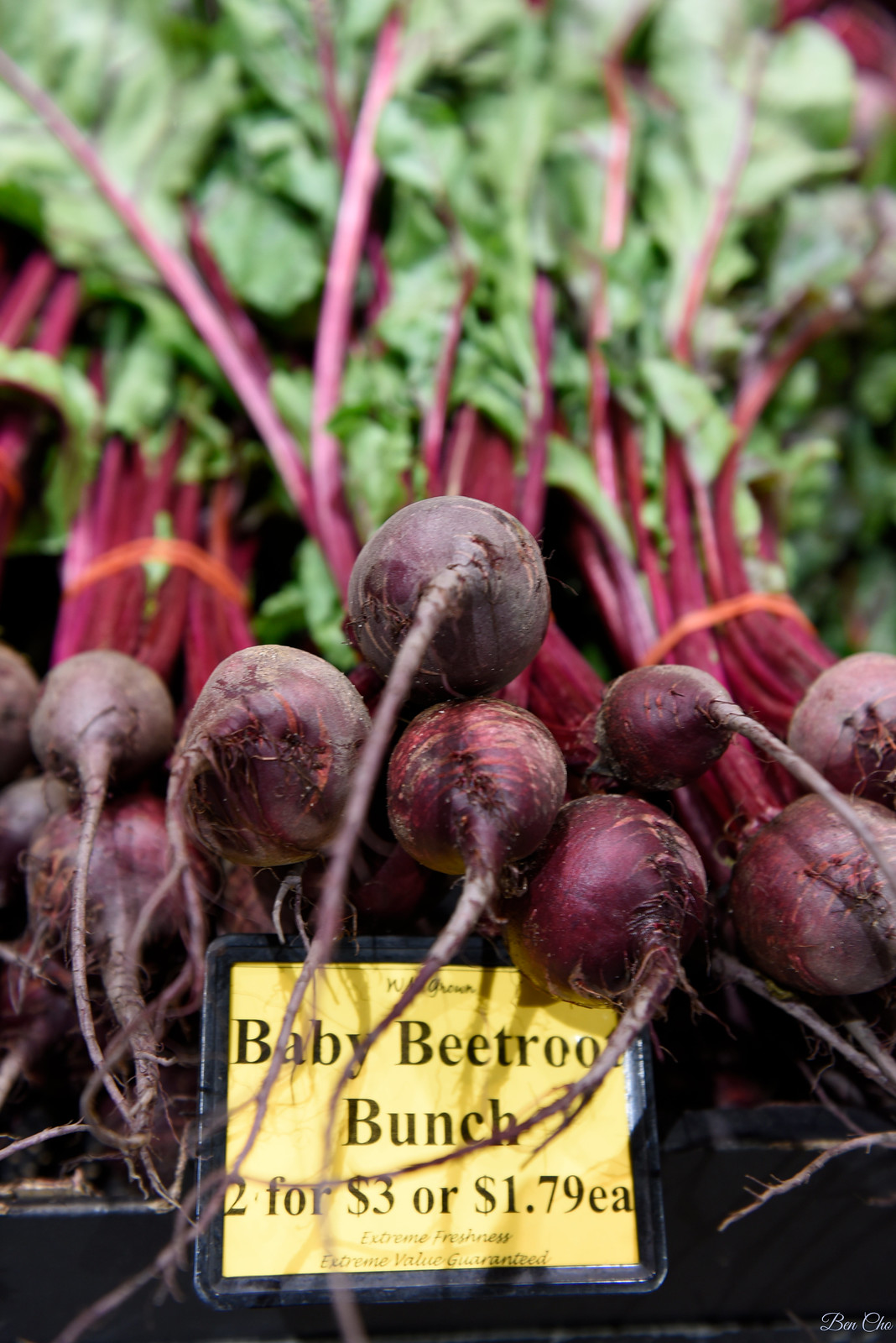The image depicts a bunch of purple baby beetroots arranged with their tips facing the viewer, laying flat and over each other. The reddish stems and green leaves are prominently seen, creating a vibrant background that becomes a bit blurry due to a bokeh effect, adding a touch of depth to the image. The front of the picture is sharply focused, highlighting a yellow price tag bordered in black and featuring bold black text. The tag reads "Baby Beetroot Bunch 2 for $3 or $1.79 each." Below the main text, smaller text states, "Extreme Freshness, Extreme Value Guaranteed." An orange band is seen binding the beetroots together. At the bottom corner of the image, there is a faint, handwritten signature, possibly saying "Bon Cha," indicating the photographer's name. The entire setup appears to be professionally taken, and the use of lighting enhances the rich colors of the beetroots.